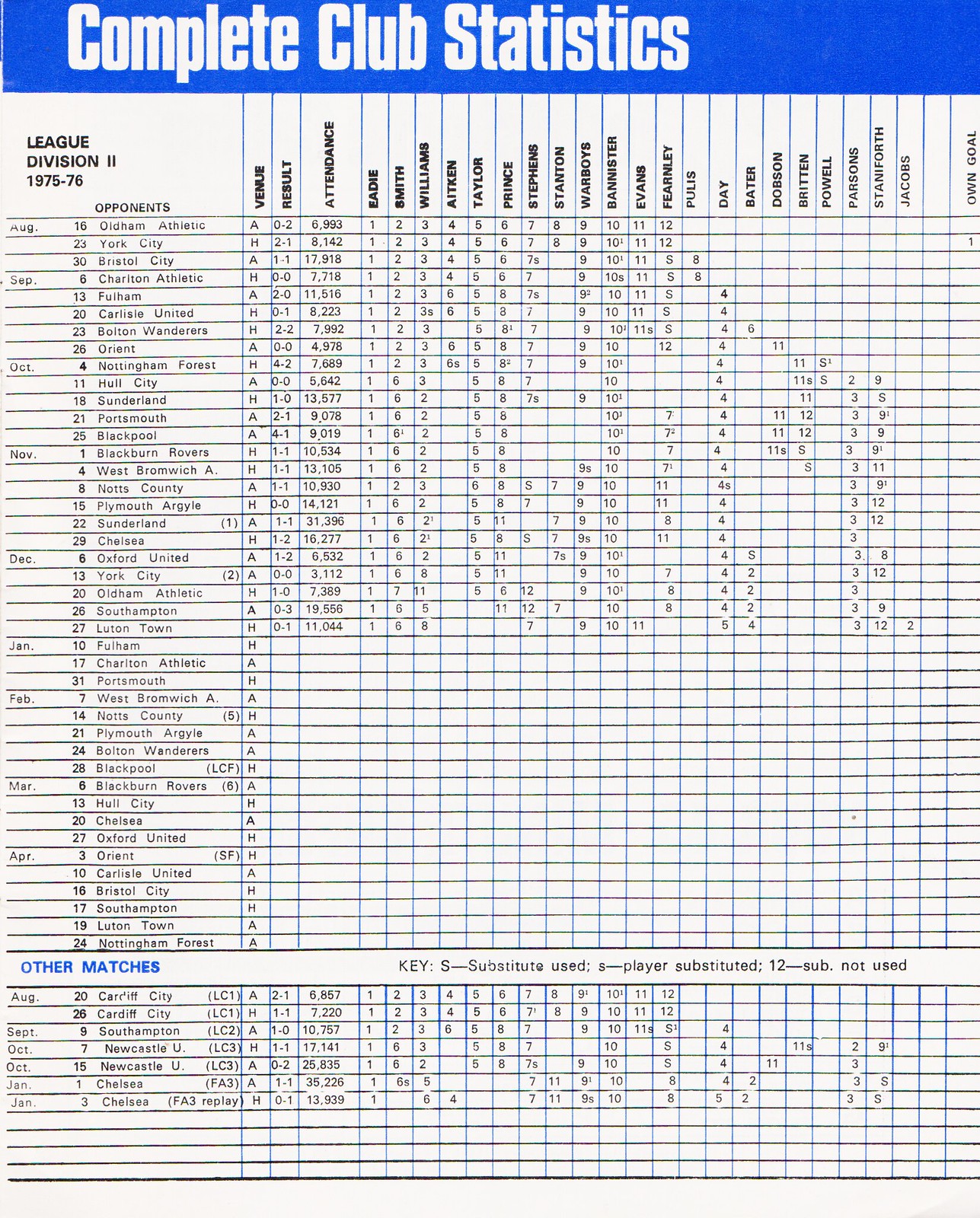The image features a detailed and comprehensive statistical chart titled "Complete Club Statistics," prominently displayed in white text on a blue rectangular header. This chart, specifically for "League Division 2, 1975-76," spans the entire page, showing a meticulous breakdown of a team’s performance throughout the season. The leftmost column lists dates from August to April, followed by a long list of opponents. Each row represents matches against various teams, detailing venues, results, and attendance. Beneath this primary section, there is another grid labeled "Other Matches" in blue, providing additional match data. The chart includes multiple columns detailing player-specific statistics, featuring names such as Smith, Williams, Atkin, Taylor, Prince, and many others. The bottom of the chart includes a key for interpreting symbols used within the data, such as "S" for substitutes.